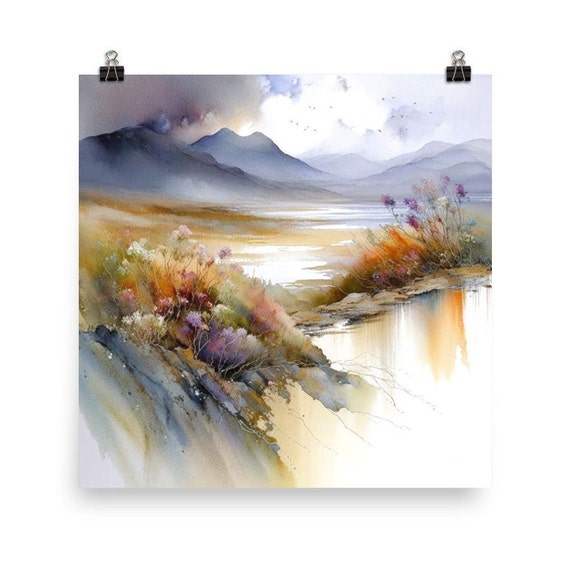This image appears to be a watercolor painting displayed vertically with black binder clips securing it at the top corners. The painting depicts a serene outdoor scene reminiscent of a desert or wilderness landscape, free of any buildings. Dominating the background are ominous mountains that transition from dark gray on the left to a light bluish-gray toward the center and right. Above, the sky features contrasting cloud coverage: dark gray clouds on the left, giving way to lighter, wispy white and gray clouds on the right with a small patch of blue peeking through the center. 

In the middle of the artwork, serving as the focal point, lies a valley or lake area that exhibits a reflective white surface—suggesting either snow or water. To the left and right of this central white space, the ground is an earthy palette of golden, brown, and orange hues, interspersed with patches of what seem to be snow or water. The bottom right section enhances the reflective quality, likely confirming the presence of water there.

Adding to the natural beauty, flowers and grasses in shades of orange, brown, and grey appear to cascade down from the left side into this white, reflective surface, evoking a sense of movement as if they are drifting or falling. The painting also subtly includes the depiction of birds soaring amongst the clouds, further enriching the tranquil and expansive ambiance of the scene.